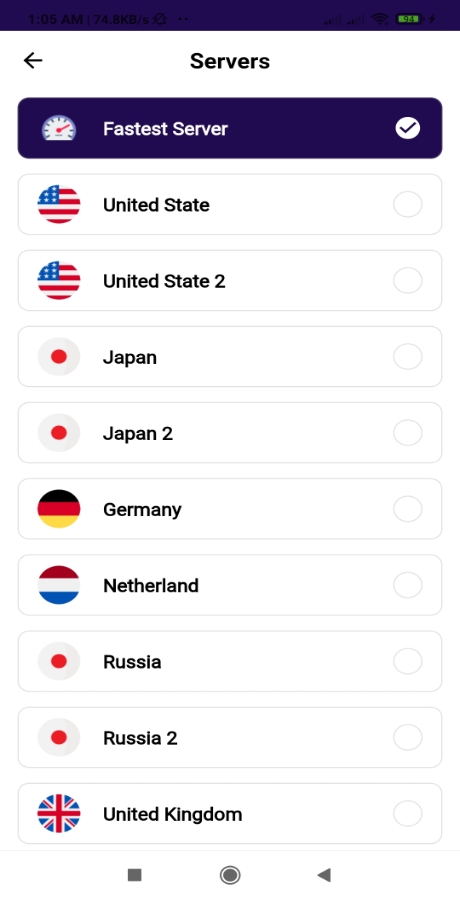The image depicts a screen displaying a list of server options for a VPN service. On the upper left side, there is a horizontal black bar with a left arrow and the word "Servers" written in black font. Directly below this bar, a highlighted server option reads "Fastest Server" in white text on a dark blue background. To the right of this option, there is a small white circle with a checkmark indicating selection.

Beneath the "Fastest Server", there is a sequence of additional server options listed by country, each with its national flag preceding it. These options include servers located in the United States, Japan, Germany, the Netherlands, Russia, and the United Kingdom. All these server options are presented within grey-outlined, long rectangles with a white background and black text. None of these options' circles are checked.

The screen features an array of colors including black, white, blue, grey, red, yellow, and green. At the bottom of the screen, typical navigation icons for a mobile interface can be seen: a square, a circle, and a right-facing arrow. Additionally, above the word "Servers," toward the top right, there is a battery icon displayed in green with a numeric indicator showing a charge level of 94%.

In total, there are ten server options visible, with nine having a white background and one highlighted in dark blue as the fastest server.